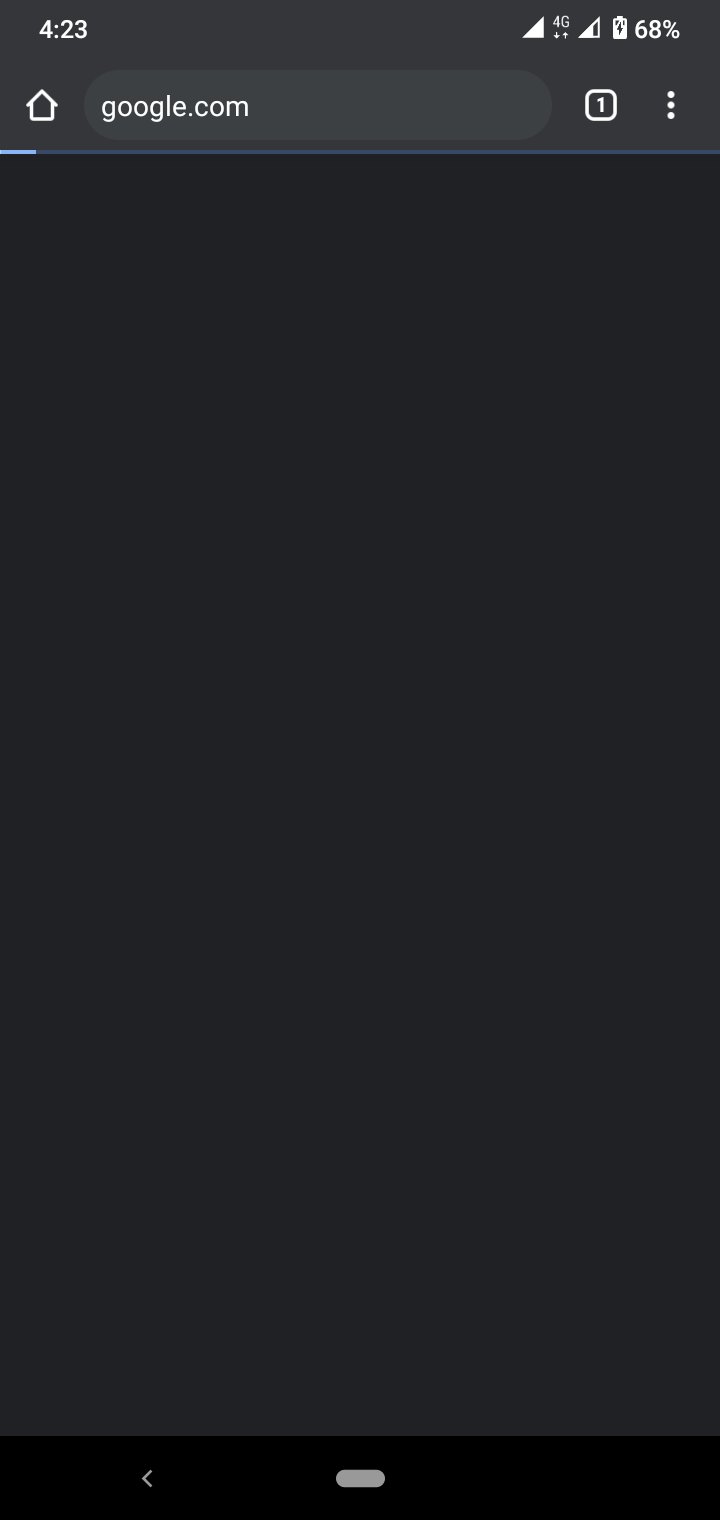The screenshot captures a live moment from a mobile device’s screen. At the very top, the status bar displays essential information: the current time is 4:23, the device is connected to a 4G network, and the battery is at 68%. The user interface exhibits a home screen icon shaped like a white house against a black, gray, and white themed background. A prominent Google search bar is located beneath the status bar, populated with the URL "google.com". Adjacent to the search bar is a small white square icon bearing the number 1, indicative of one unread notification or tab. Following the square icon are three vertical dots, signifying additional options or settings. Just below the search bar, a thin blue line indicates that the web page is actively loading. The remainder of the screenshot is predominantly black and unoccupied, suggesting the page content has yet to appear or further loading is required.